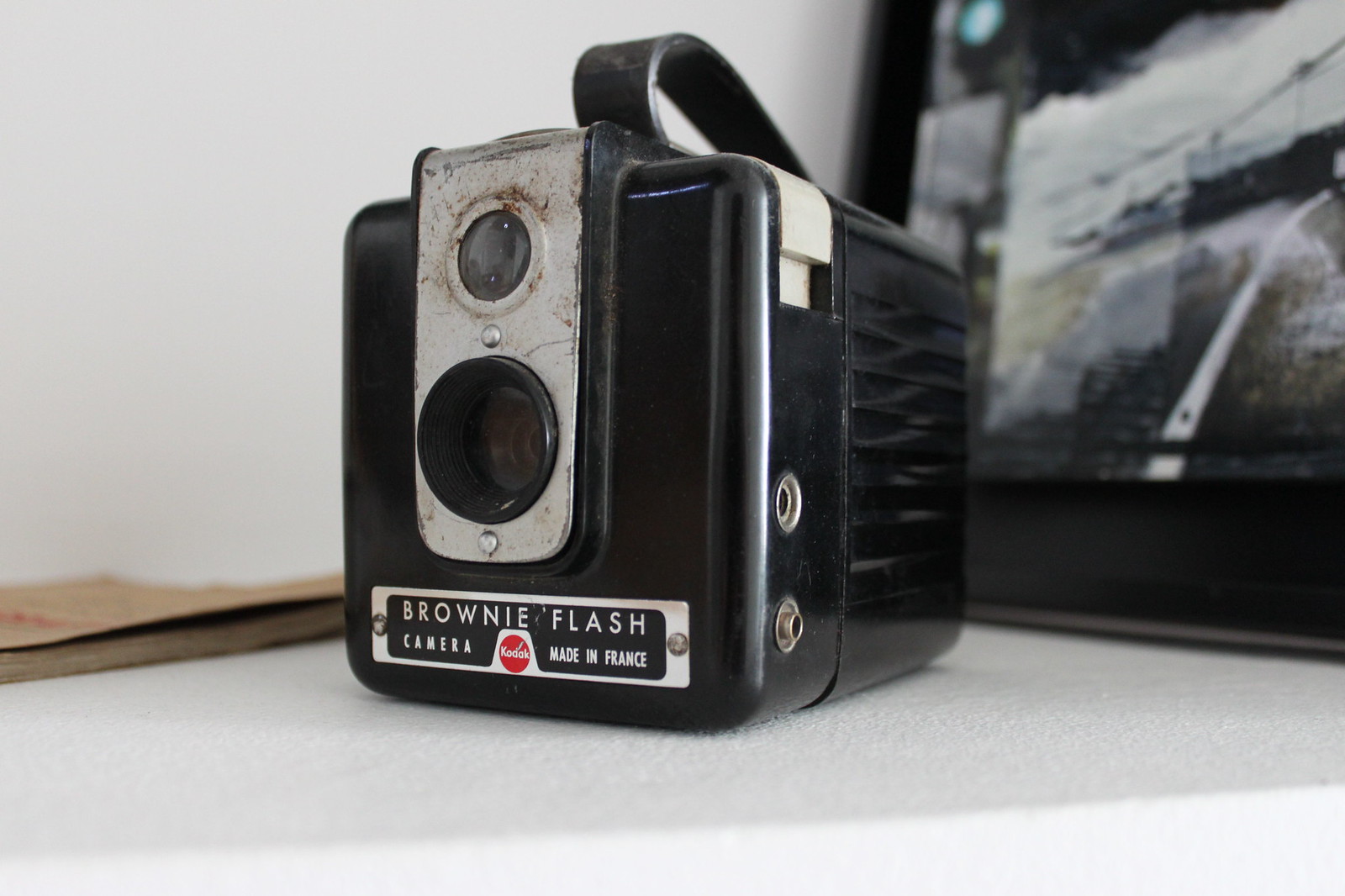This close-up photograph, taken indoors, showcases an old-fashioned Brownie Flash Camera, made in France. The camera, almost cube-shaped and black in color, stands prominently on a white counter. Its vintage design features a slightly tapered front with a gray panel down the center, displaying two glassy lens areas—one with a small black cylinder or funnel. Accentuating its nostalgic charm, the camera bears visible wear, with a scratched and slightly rusted metal piece near the lens. The top hosts a curved black leather handle, and below the lens area is a bolted-on metal placard that reads, "Brownie Flash Camera, Made in France," complete with a red company logo. The right side of the camera has two small portholes, likely for connections. The background reveals a white wall, a potential manual or book to the left, and an indeterminate framed image to the upper right.